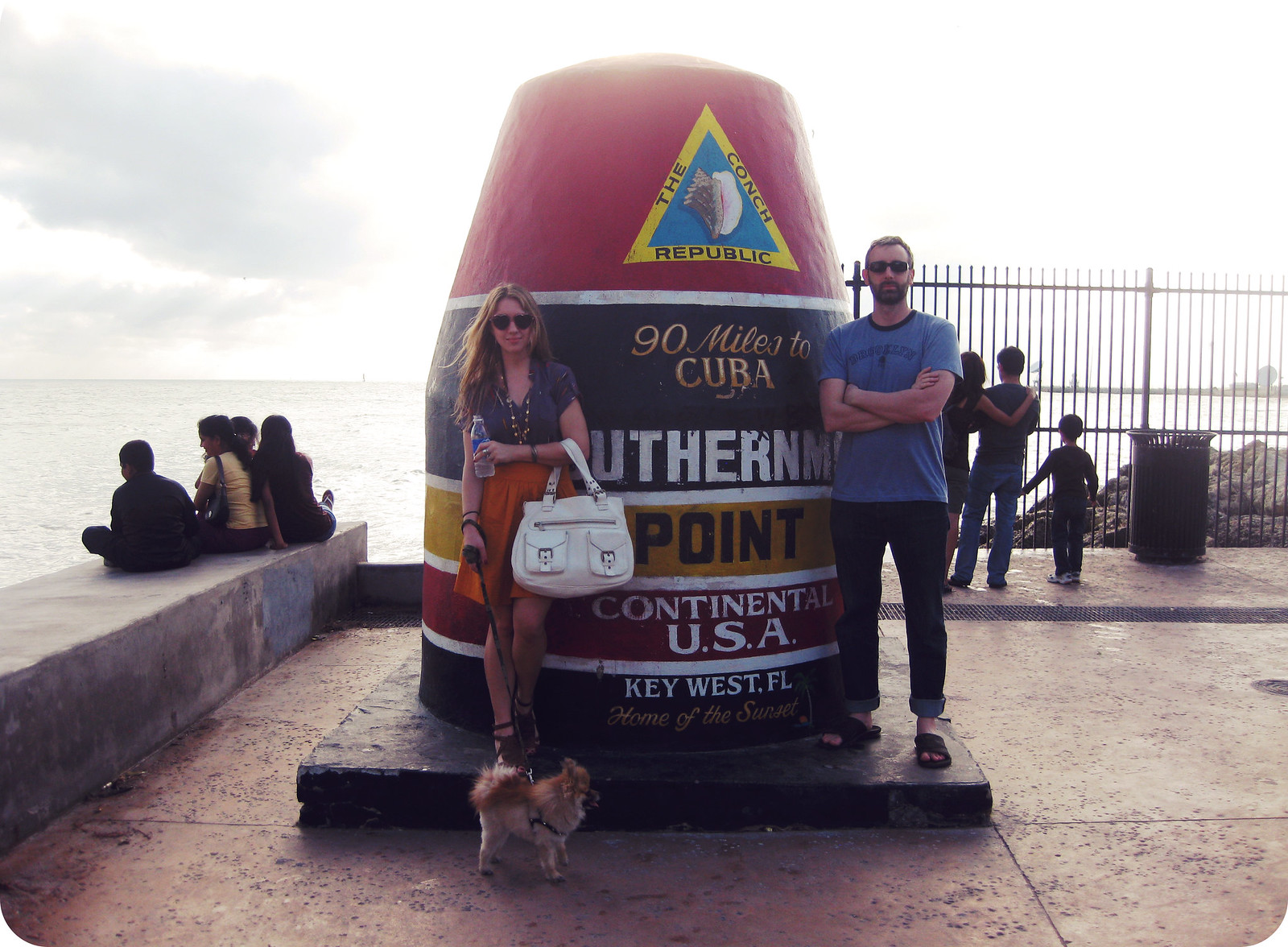This photograph captures the southernmost point of the continental United States, located in Key West, Florida, right next to the ocean. At the center of the image stands a large, multicolored buoy-shaped monument that reads: "90 Miles to Cuba, Southernmost Point, Continental USA, Key West, Florida, Home of the Sunset." The monument features a distinctive color scheme with bands in black, yellow, and red, and a triangular emblem at the top sporting the words "The Conch Republic."

Two individuals, a man and a woman, are prominently positioned in front of the monument, appearing to be tourists. The man, wearing a blue t-shirt and blue jeans, stands a foot taller than the woman, who is dressed in a gray shirt, orange skirt, and carries a white purse. The woman also holds the leash of a small brown dog. Both individuals wear sunglasses, and they are standing on the black pedestal that supports the monument.

In the background, the ocean and a gray seawall are visible. To the left, four people are seated on the ledge of the seawall, mostly dressed in black clothing with one person in blue jeans. To the right, another group of three people, including a woman, a man, and a child, are standing along a metallic black fence. The man wears a blue shirt and blue jeans, similar to the central male figure, and the child is dressed in all black.

Further right, some gray rocks and a black garbage can are noticeable. The entire scene exudes a commemorative atmosphere, capturing a popular tourist spot marked by the unique monument indicating the southernmost point of the continental U.S. with its iconic "90 miles to Cuba" inscription.